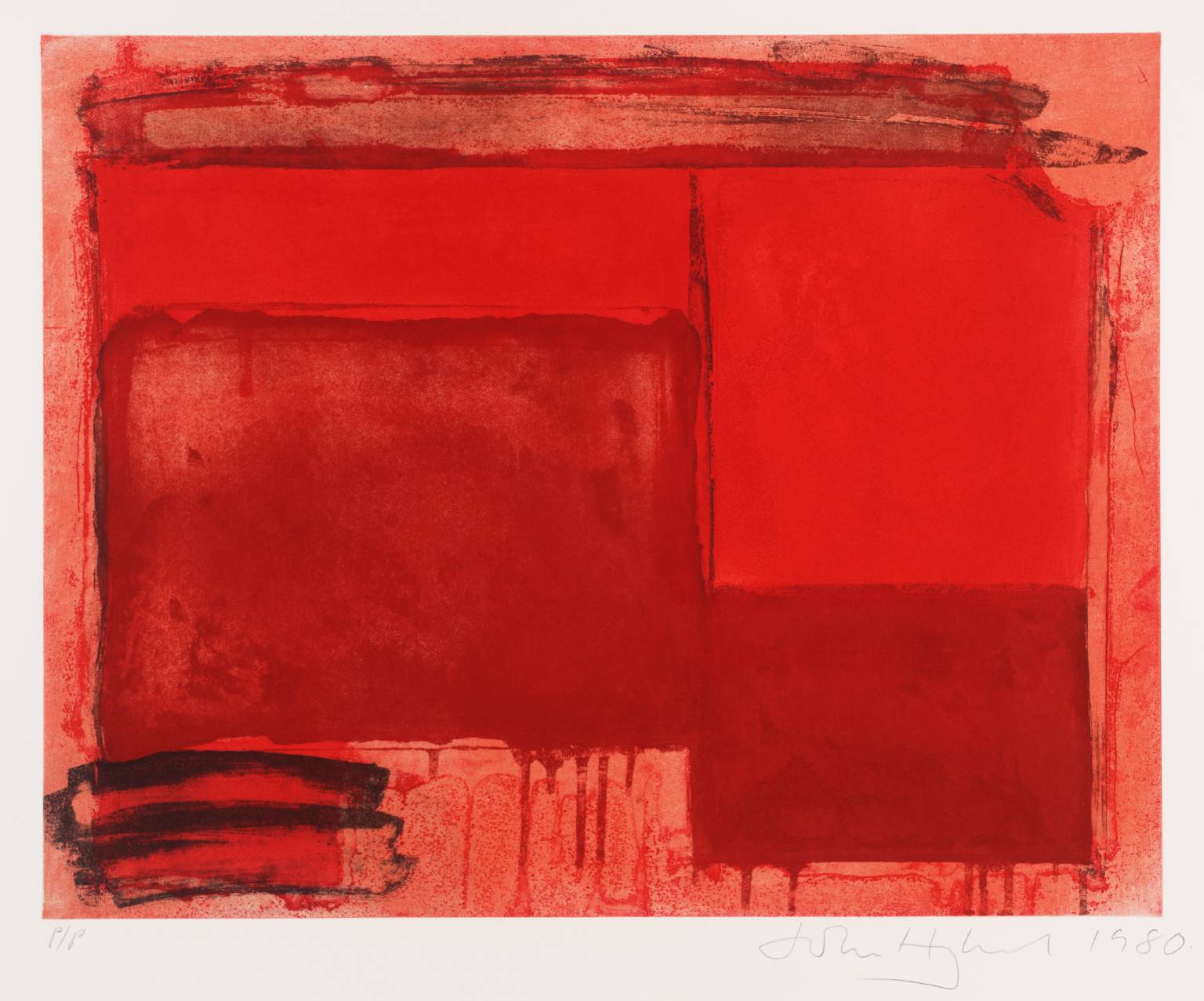The image illustrates an abstract painting that prominently features various shades of red. Dominating the composition, a vivid red background serves as the canvas with a distinct horizontal red line running across the top. Near the top, the red begins to blend into softer pink hues, adding depth and variation to the piece. Central to the painting are two maroon-colored rectangles: a larger one positioned in the middle left and a smaller one situated in the bottom right corner, approximately half the size of the larger rectangle. These maroon blocks exhibit a slight bleeding effect where the paint appears to be running downward. Below the larger maroon rectangle, in the lower left-hand corner, there are two distinctive black smudged lines stacked on top of each other, lending a sense of texture and contrast. Additionally, lighter red rectangles, one directly above the larger maroon block and another brighter red rectangle encompassing about three-quarters of the painting's central area, add complexity to the overlapping structure. The top section of the image is adorned with abstract swishes and drips, where the colors blend seamlessly into the background. The piece, framed with an understated border, is signed "John Hughes 1980" at the bottom, marking its creation year.